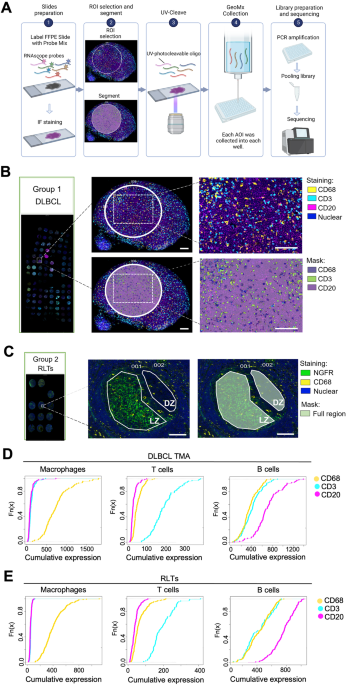This image appears to be a detailed scientific diagram, likely from a textbook or a presentation. It is structured into five rows labeled A through E. 

- **Row A** features five rectangular images detailing the preparation of a slide, possibly indicating various stages or different techniques used.
- **Row B** contains four images, each offering a microscopic view of an unidentified substance, with vibrant colors suggesting diverse features or treatments.
- **Row C** displays two detailed images, also apparently microscopic views of a substance, continuing the pattern of detailed observation.
- **Rows D and E** each present three charts with red, green, and yellow lines trending upwards from the lower left to the upper right corners, indicative of data measurements. These graphs likely represent the behavior of different infused waters under certain conditions, showing how each type evaporates over time.

The collective emphasis on microscopic imagery and graphs suggests this diagram pertains to a study on how various substances react to thermal processes, possibly explaining the mechanics of a thermal device used for heating or evaporating liquids. The colorful and detailed visuals imply a deep investigation into the characteristics and behaviors of the substances under study.